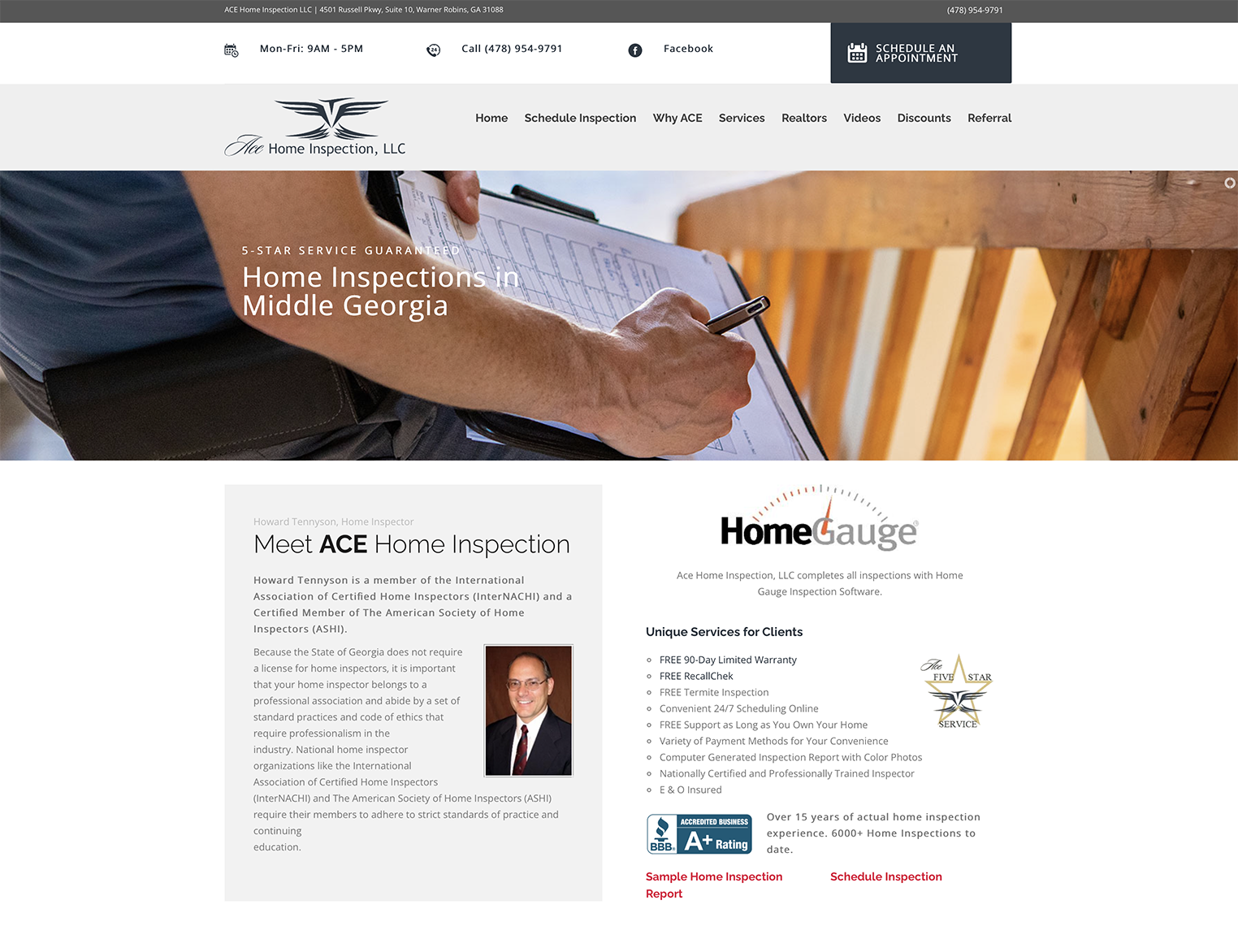The image is a screenshot from a webpage designed for viewing on smart devices or desktop screens. The background of the webpage is predominantly white, utilizing the default white of the computer screen.

At the very top, there is a long, dark gray rectangular bar. On this bar, inset slightly from the left, the text "ACE Home Inspection, LLC" is displayed in white. Accompanying this is the company's address in Georgia. Towards the right side of this bar, but still within the page’s central area, the phone number is listed.

Beneath this, positioned to the left, there is a small calendar icon indicating the business hours: Monday through Friday, 9 a.m. to 5 p.m. Adjacent to this, there's an option to call the company, along with a Facebook icon for social media access. Further to the right is a dark blue rectangular button featuring a calendar icon and the text "Schedule an Appointment."

Below these details, another gray bar features the company's logo and the name "ACE Home Inspection, LLC." Following this are clickable options: Home, Schedule Inspection, Why ACE, Services, Realtors, Videos, Discounts, and Referral.

The primary image showcases a man's arm and hand holding a checklist, actively writing on it. This is accompanied by the text, "Five-Star Service, Guaranteed Home Inspections in Middle Georgia."

Further down, the page introduces "Howard Tennyson, Home Inspector" with a profile picture and a brief bio about him. To the right of this, a "HomeGauge" logo is displayed, highlighting "Unique Services for Clients." The list includes credentials like the A+ rating from the Better Business Bureau (BBB) and emphasizes their five-star service.

Prominently in red text, the webpage offers links to a "Sample Home Inspection Report" and a "Schedule an Inspection" option for further interaction.